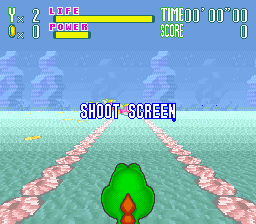This image is a low-resolution screenshot of a square, digital video game designed for children. The game interface is divided into two main sections: the top half features a sky-blue backdrop, while the bottom half showcases a green terrain interspersed with brown mountains or earth formations that converge towards the center from the bottom corners. Dominating this lower portion is a dinosaur-like creature, identifiable by the row of spikes along its back. The dinosaur, with a green head, gazes towards the foreground. Above the dinosaur, bold, white uppercase text outlined in blue commands the player to "SHOOT SCREEN." In the foreground beneath this text, several indistinct characters add to the scene, their details blurred by the image's low resolution.

At the top of the screen, a user interface bar with pink and yellow hues displays the player's life and power levels. Additionally, the top right corner includes sections for tracking the in-game time and score. The overall color palette harmoniously blends soft light blue, green, and bright yellow tones, contributing to the game's inviting and playful aesthetic.